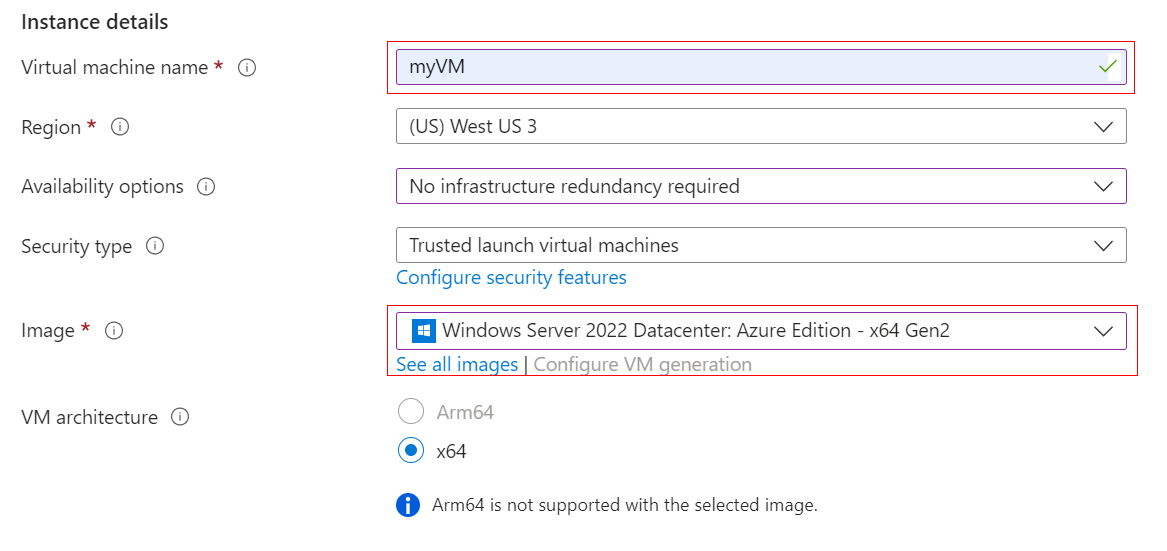The image depicts a virtual machine setup interface within a Windows operating system, presented against a white background. In the top-left corner, "Instance Details" is prominently displayed. Below this heading is a list of required selections for setting up the virtual machine.

The first entry requires the "Virtual Machine Name," indicated by black text and an accompanying red star, signifying a mandatory field. Adjacent to this label is an information icon enclosed in a circle. The name entry field, outlined in red, contains the text "My VM."

The next field is "Region," also marked with a red star. It specifies "US (West US 3)," indicating the required input. This is followed by "Availability Options," which reads, "No infrastructure redundancy required."

The "Security Type" section lists "Trusted launch virtual machines," with a link below in blue text reading "Configure security features."

The "Image" section, another mandatory field marked by a red star, also has its selection box outlined in red. The selected option is "Windows Server 2022 Data Center Azure Edition x64 Gen 2." Below this selection, a blue text link states, "See all images."

A vertical black line labeled "Configure VM generation" in gray separates the next sections. Lastly, under "VM Architecture," users can choose between "ARM64" and "x64." A blue circular icon with an exclamation mark indicates that "ARM64 is not supported with the selected image."

This detailed depiction ensures a comprehensive understanding of the virtual machine setup interface.